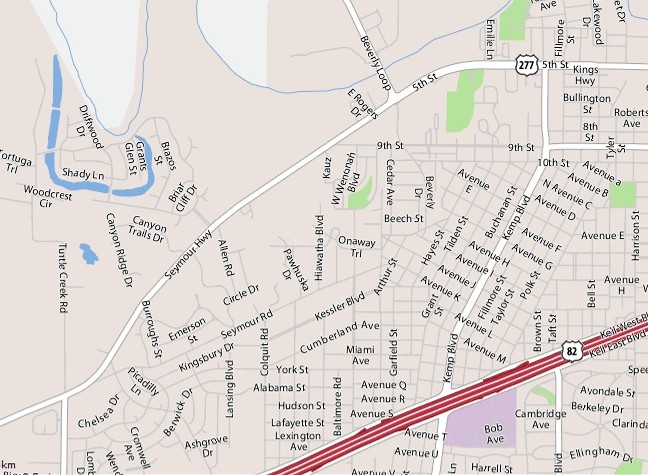The image showcases a detailed map featuring numerous street names. In the bottom corner, there are three prominent red strips, each adorned with a shield emblem displaying the number "82." This section highlights Cal East Boulevard and Cal West Boulevard, both running parallel in the same stretch. Moving towards the top of the image, another major road is visible, marked with the same shield emblem and the number "277." This road, identified as 5th Street, traverses the map from left to right. As it extends to the left, 5th Street curves downward and forks off to the right into an area labeled Beverly Loop. Continuing from this junction, 5th Street transitions into Seymour Highway. The map also features blue areas indicating bodies of water, which are surrounded by various streets, including Shady Lane, Woodcrest Circle, Grants Glen Street, Driftwood Drive, and Canyon Ridge Drive.